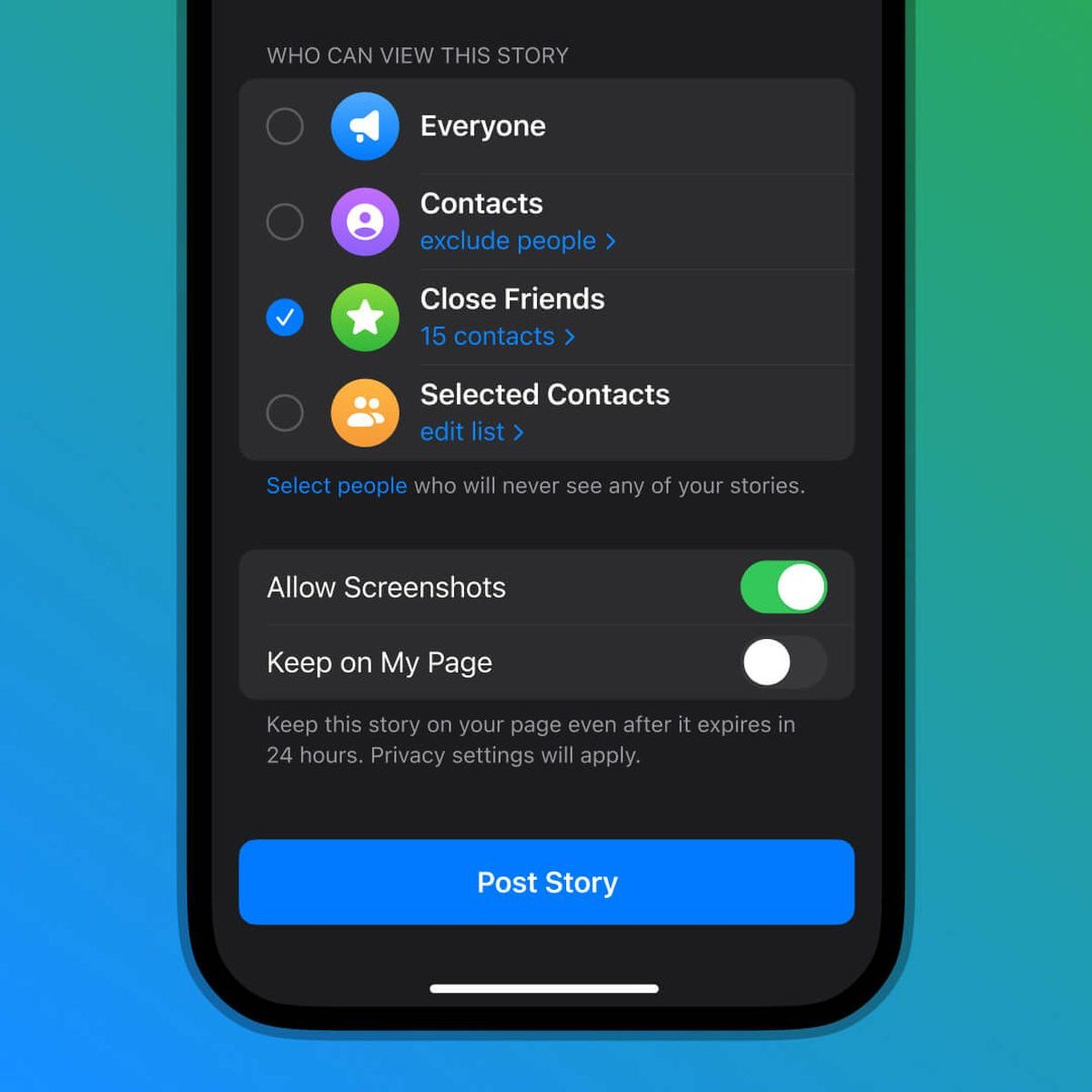This screenshot displays the lower half of a cell phone, showcasing part of both the device's exterior and its active screen. The screen content pertains to setting privacy options for a story, with the heading "Who can view this story." Below this heading, there is a black box containing four distinct privacy options, each accompanied by an icon and descriptive text.

1. **Everyone**: Represented by a blue circle with a white megaphone icon. This option is unselected.
   
2. **Contacts**: Displayed with a purple circle containing a white person icon. Below "Contacts," there is an additional blue link labeled "Exclude people." To the left, an unselected option with a person icon is shown.

3. **Close Friends**: Indicated by a green circle with a white star. This option is currently selected, denoted by a blue circle with a white checkmark. Below "Close Friends," it mentions "15 contacts" with an arrow pointing to the right.

4. **Selected Contacts**: Illustrated by an orange circle with an icon of two people. This option is unselected. Below "Selected Contacts," there is a blue link labeled "Edit list" with an arrow pointing to the right.

Beneath this black box, there's a prompt that reads "Select people who will never see any of your stories." Following that, there are two toggle options:

- **Allow screenshots**: This toggle is switched on, marked by a green indicator.
- **Keep on my page**: This toggle is switched off.

At the bottom of the screen, there is a prominent blue button labeled "Post Story."